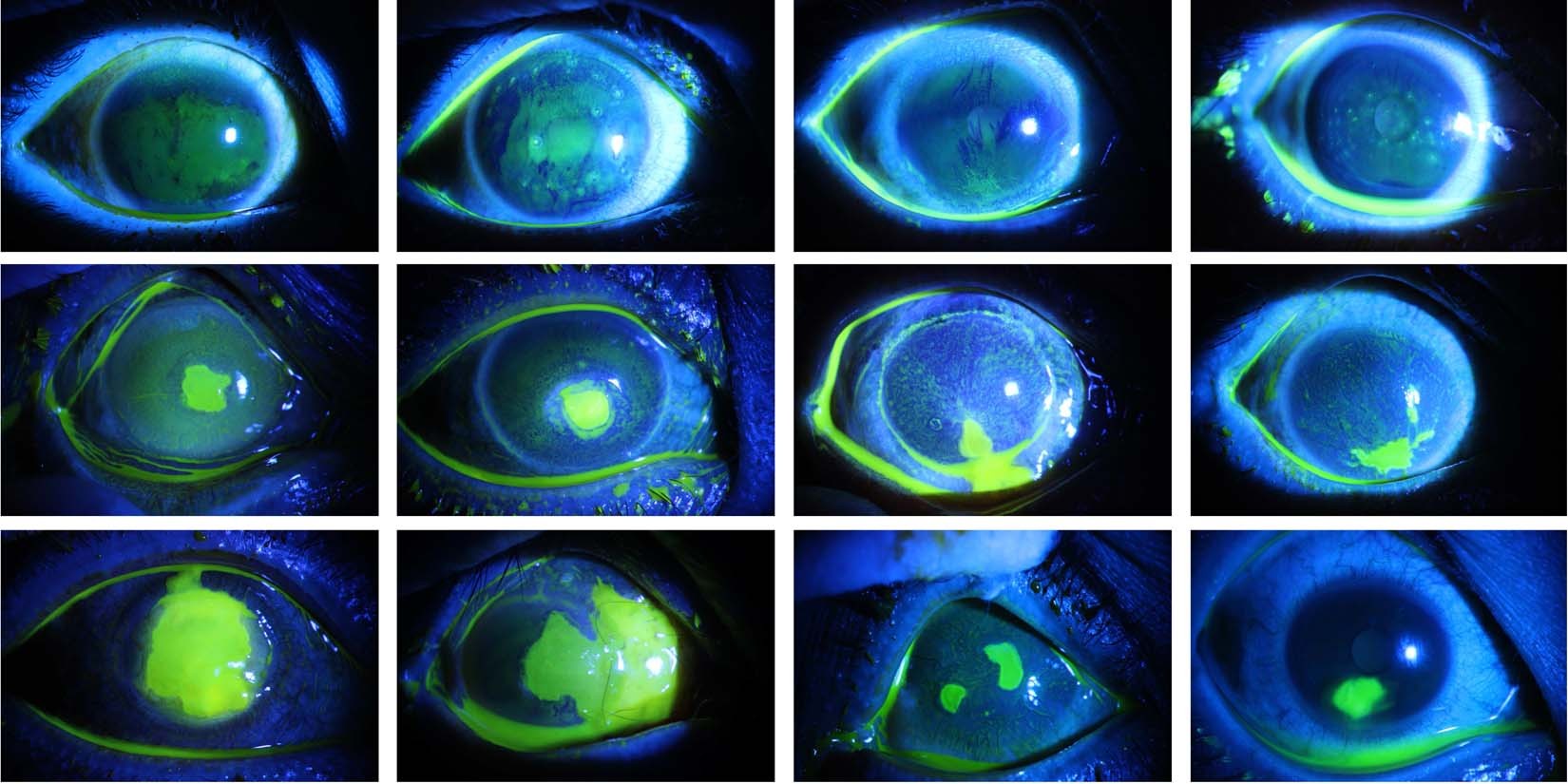The image is a rectangular grid comprising 12 close-up photographs of eyes, arranged in three horizontal rows of four. Each eye photograph has a stark black background, enhancing the vivid colors of the irises. The majority of the eyes are predominantly blue, with varying amounts of green and neon yellow splattered throughout. 

Notably, the first eye in the upper left corner features a blue outer lining with a misty green and a hint of blue in the center. The adjacent eye to the right displays a green strip in the upper left with blotchy green in the middle, surrounded by blue. In the bottom right corner, the eye has a dark blue center with a distinctive green blotch near the bottom and a green line below the iris. The eye next to this one showcases two prominent green blotches amidst a blue background.

Each eye appears moist and squishy, with some images showing a wide-open iris. One eye in the lower right corner stands out, resembling a human eye with a visible white sclera that appears bloodshot and an eyelid partially in view. The vibrant reflections, possibly from a blue light shining on dyed eyes, create a compelling array of green hues against the blue, highlighting the variation in green dye applications. Overall, these eyes evoke a sense of both commonality and unique details across the series.